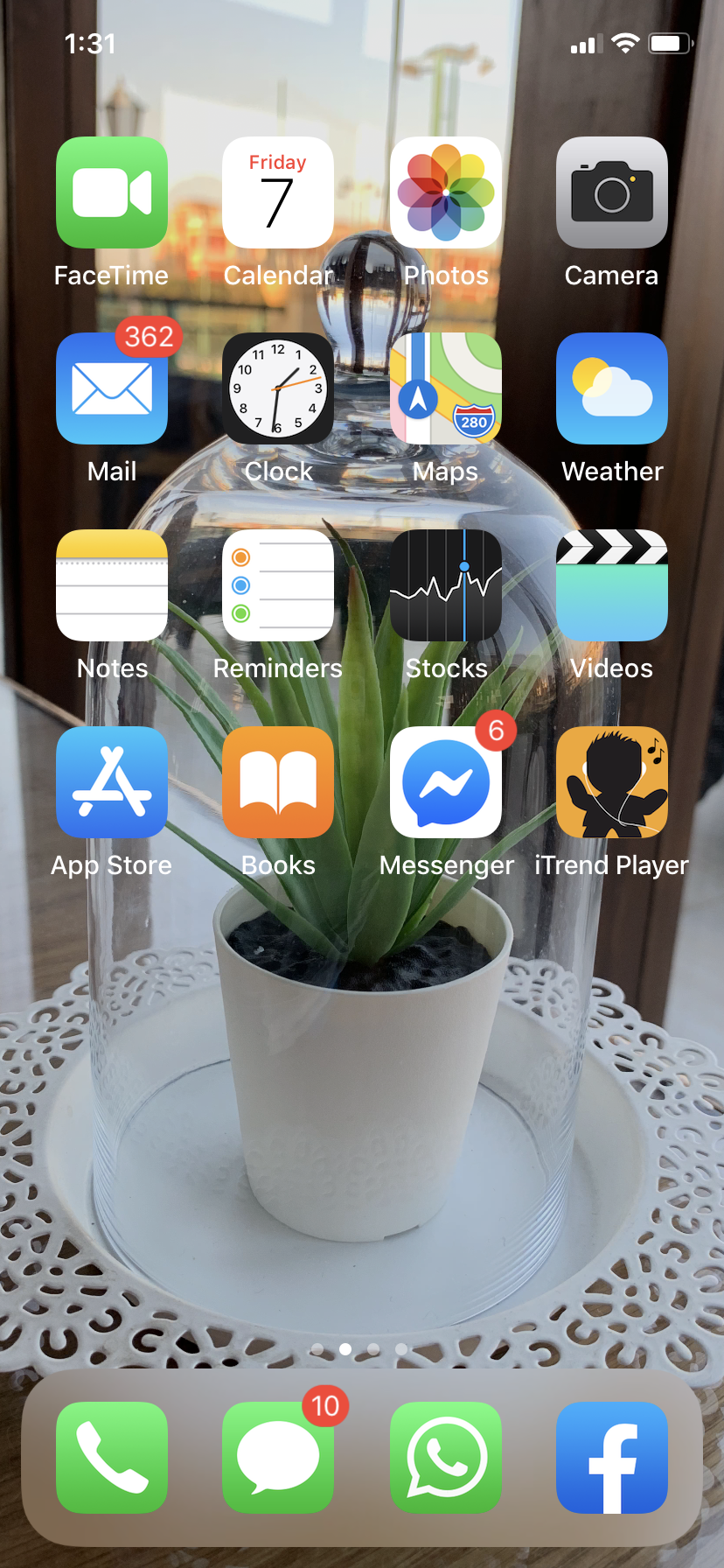This detailed screenshot captures the homepage of an Apple phone. The backdrop features an artistic photograph showcasing a serene tabletop scene. At the center, a delicate doily lays spread out, upon which rests a pristine white plate. On the plate sits a petite white cup, cradling a lush jade plant rooted in rich, dark soil. A sophisticated clear glass bell cover encases the plant, adding a touch of elegance. The backdrop of this image presents a softly blurred cityscape viewed through a window, imparting a tranquil ambiance.

The phone's homepage is populated with various app icons, neatly arranged. Notable icons include FaceTime, Calendar, Photos, Camera, Mail, Clock, Maps, Weather, Notes, Reminders, Stocks, Videos, App Store, Books, Messenger, and iTrend Player. Along the bottom banner, quick-access buttons for Phone, Messages, Voicemail, and Facebook are prominently displayed, ensuring easy navigation for the user.